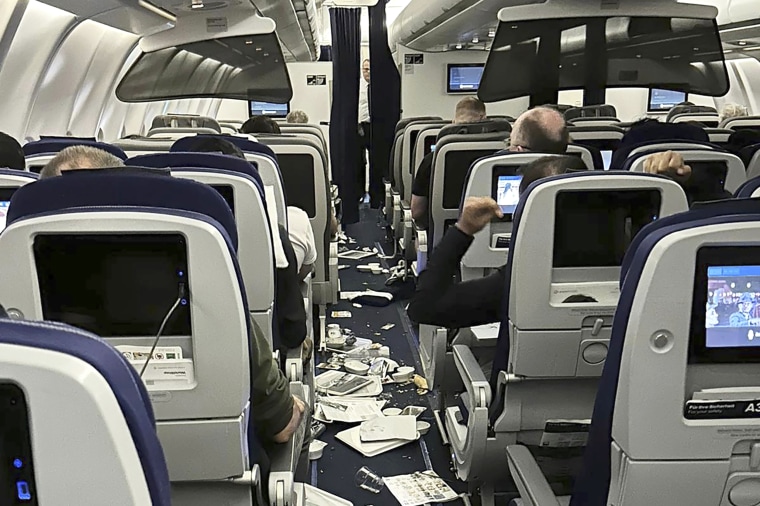This is a photograph taken from the rear of an airplane's passenger section, capturing the view down the aisle towards the cockpit. The seats, which appear to be a light tan or off-white color, rise in neat rows with the tops of passengers’ heads visible—some with dark brown hair and one noticeably balding. A dark gray carpet runs along the aisle, currently strewn with debris such as papers, cups, trays, and crumbs, suggesting recent turbulence may have caused items to fall. Small screens are embedded in the seat backs, mostly black but with a couple showing content being watched. Near the front of the cabin, black curtains partially obscure the galley area, through which an airline employee—dressed in a white shirt, black tie, and black pants—peers with half of his face visible. Everyone remains seated, some with tablets in use, continuing their journey amidst the scatter of items in the aisle.